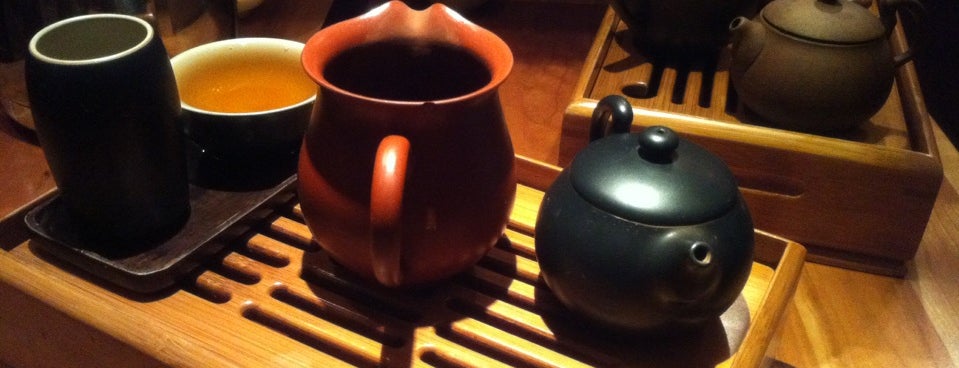This image showcases a rustic tea setting arranged on a light-stained wooden table with matching TV trays. The nearest TV tray, crafted from the same light wood, features a smaller dark wooden tray that holds a black coffee mug with a white or silver interior, paired with a matching black bowl. Centered on this TV tray is a vibrant red pot, while an additional blue pot is placed at the upper right corner. The second TV tray, situated farther back, supports a brown pot, barely visible in the dim, warm lighting. On the left side of the scene, there’s a brown wooden tea container and a black kettle, framed by soft shadows, creating a cozy, inviting atmosphere. The detailed arrangement of teapots and cups, paired with the warm lighting, evokes a sense of serene, relaxed tea time.